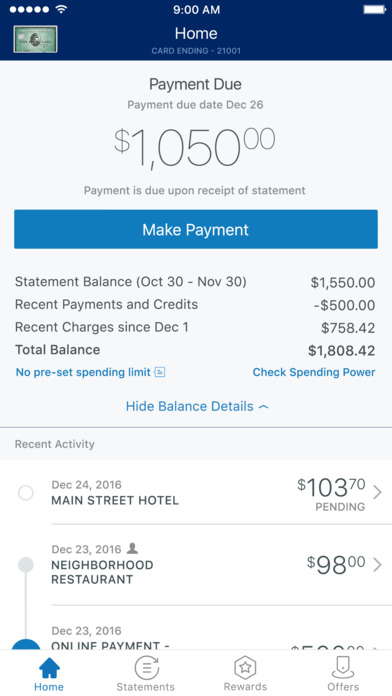The image showcases a detailed screenshot of an American Express account statement. 

In the top left corner, there are standard smartphone status indicators: five white circles, indicating full Wi-Fi signal, the time displayed as 9:00 AM, and a full battery icon. Below, the statement header includes details about the American Express card, specifying that the card ends in 21001. The due date for the payment is December 26th, with a due amount of $1,050. A blue rectangular button labeled "Make Payment" is visible below the payment details.

Further down, the statement balance for the period from September 30th to November 30th is indicated as $1,550. This balance is adjusted with receipts and credits, showing a deduction of $500, and subsequent credits since December totaling $758.42. The total outstanding balance is noted to be $1,800.42. There is no preset spending limit, and a prompt to "Check Spending Power” is included.

Recent transactions are listed with dates and details: 
- On December 24th, 2016, a charge of $903.77 at Main Street Hotel.
- On December 23rd, 2016, a $98.00 charge at Neighborhood Restaurant.
- Also on December 23rd, 2016, an online payment.

At the bottom left of the image, navigation buttons are visible: "Home," "Statements," "Rewards," along with a set of numbered circles from 1 to 48, likely pagination indicators or additional navigation options for account management.